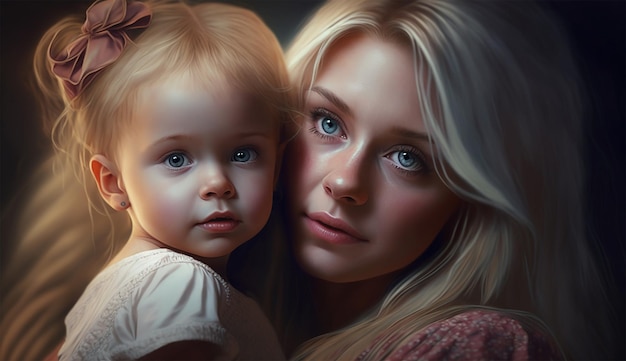This digital rendering presents a heartwarming portrait of a mother and child. The mother, placed on the right, has long, cascading blonde hair and strikingly big blue eyes. She dons a pale pink shirt and holds her young daughter closely. The child mirrors her mother's features with similarly beautiful blonde hair adorned with a pink bow, big blue eyes, and rosy lips. She is dressed in a white shirt featuring a delicate design. Both appear to have porcelain-like skin, smooth and flawless, exuding a soft and gentle tone. The background is a deep black, enhancing the lifelike quality of the artwork and focusing attention on the intimate bond between the two. They both gaze directly at the viewer, further drawing them into the serene and touching scene captured by the artist.